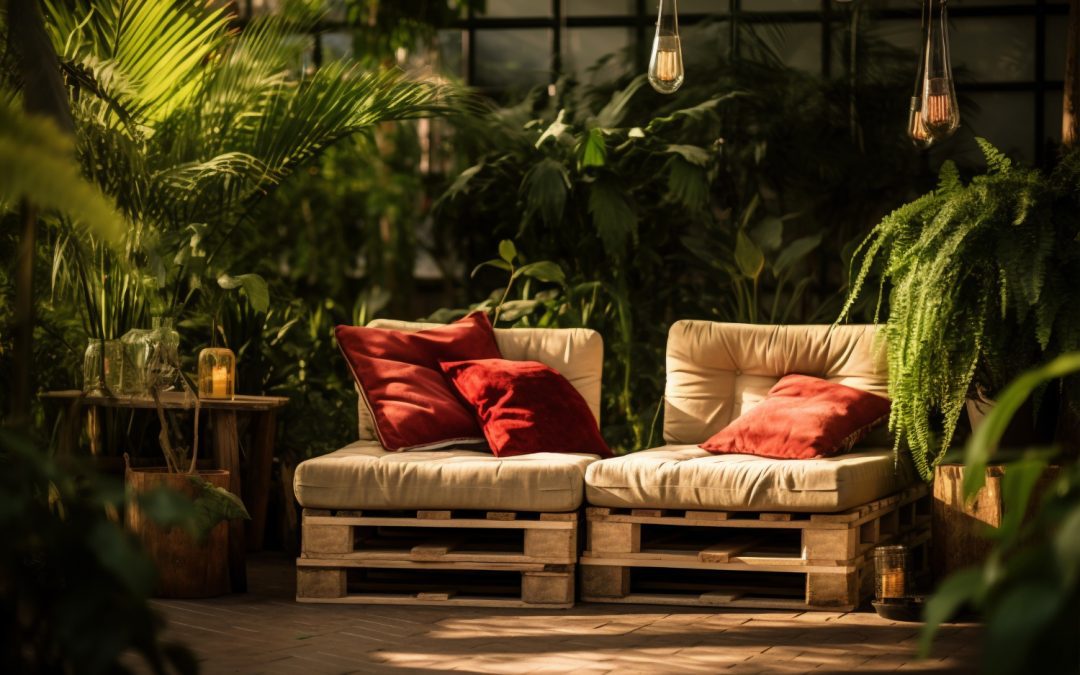In this horizontally-oriented photograph, we see two lounge chairs crafted from stacked wooden pallets, now transformed into cushioned seating. Each chair features large beige cushions with a white backrest, and they are adorned with vibrant red throw pillows—two on the left chair and one nearly flat on the right chair. The scene seems to be set in an outdoor area like a patio or porch, although it could also be inside a solarium. The floor consists of tan-colored bricks, adding to the rustic charm of the space.

The chairs are framed by abundant greenery, with large, tropical plants like palm fronds and ferns surrounding them. Notably, a fan palm is visible to the left of one of the chairs. Behind the seating area, glass windows suggest the presence of an adjacent room that allows for an unobstructed view of the garden-like setting. Sunlight from the left casts a warm, dappled glow over the chairs and highlights a table with a candle beside them, suggesting a serene time of day, possibly dusk. This harmonious blend of natural elements and cozy, repurposed furniture creates an inviting and tranquil outdoor retreat.